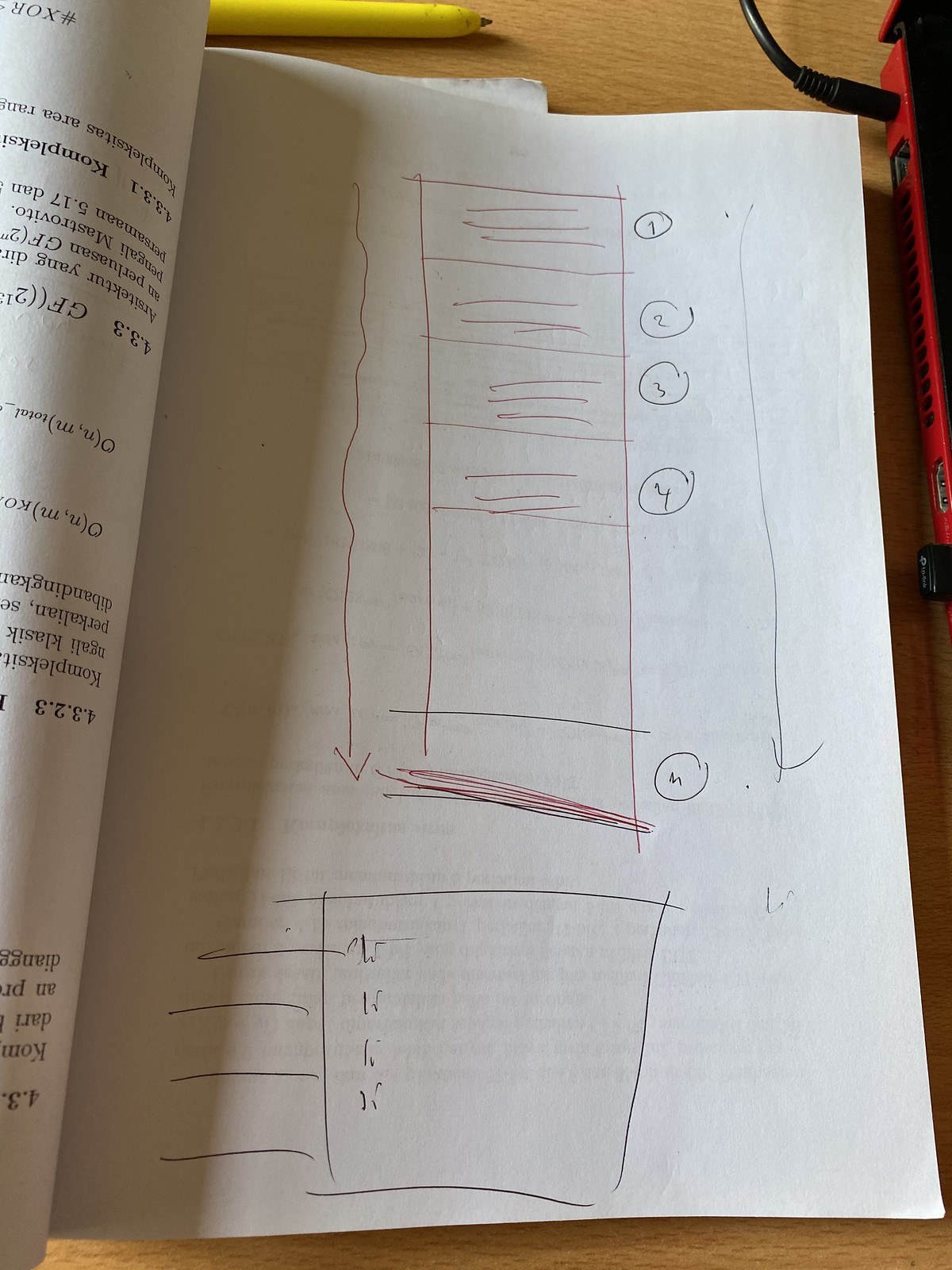An open notebook lies on a brown desk, captured in a close-up shot that reveals intricate details. The notebook’s white pages contrast starkly against the rich brown of the wooden surface. At the top of the image, a pencil rests horizontally on the open pages. To the right, you can spot the edge of a laptop with a cord plugged into it, adding a touch of modernity to the otherwise simple scene.

The notebook's left page is filled with handwritten notes in two distinct sections. The top section is marked with a red pen, featuring a large vertical rectangle divided by horizontal lines. Numbered steps, "1" through "3", are encircled and accompanied by a large downward-pointing arrow, suggesting a sequence or progression. This section appears to be an outline or a schematic for an idea or project, though its exact purpose isn't definitive.

The bottom section of the page, written in black ink, shows a large square also divided by horizontal lines. Each line is marked with the number "1", repeated four times. This seems to indicate a structure for organizing information, potentially designating four main points or headings to be expanded upon later.

The image, with its mix of handwritten notes and digital tools, captures a moment of planning and creativity in progress.